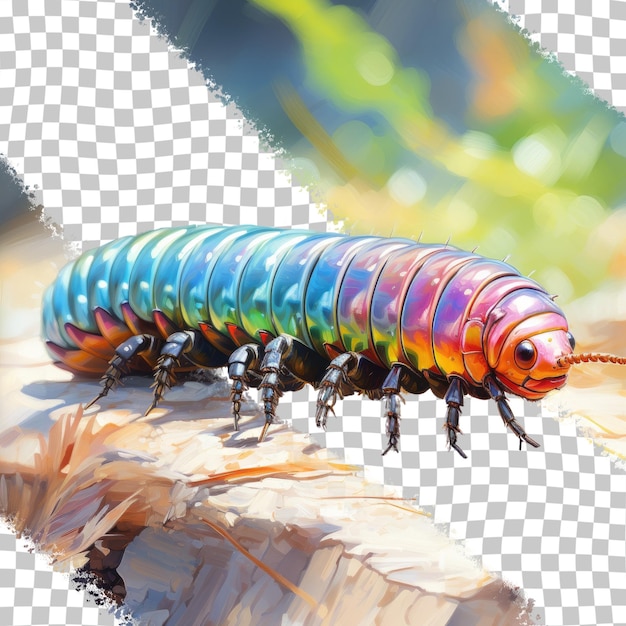This image is a detailed, computer-generated artwork focused on a centipede. The vertical rectangular composition features the centipede prominently within a blurred, green-tinted background. There are distinctive white stripes adorned with gray diamonds running horizontally across the image from the top right to the bottom left. 

At the center of the picture rests a tan rock from which the metallic-looking centipede emerges. It transitions through various colors along its segmented body: starting with a grayish-silver near the middle, moving towards teal blue, then transitioning to light blue, purplish-pink, orange, and finally reaching its head. The centipede has numerous black legs on each side, with eight or nine visible along the right-hand side, and two large black circular eyes positioned at the head, which is oriented towards the right. 

The intricate color palette includes light green, yellow, light blue, dark blue, light pink, orange, light purple, gray, tan, beige, and off-white, emphasizing the artist's detailed approach to rendering the centipede. The image does not contain any text or words, highlighting the centipede's vivid, multicolored appearance and artistic representation. The overall effect is an engaging, detailed portrayal of a centipede within a stylized, computer-generated setting.